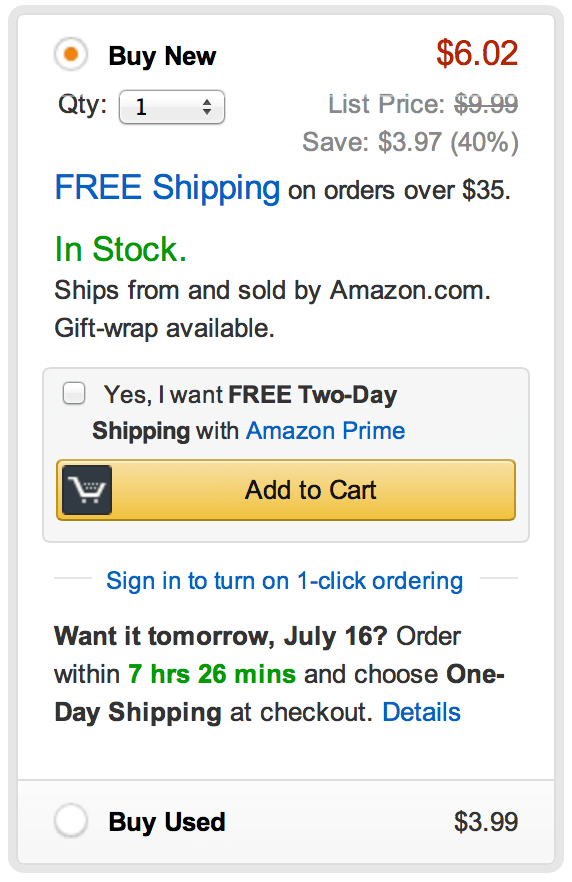The image showcases a mobile phone screen displaying an Amazon product page. Key elements include a prominent "Buy New" option highlighted in black text. To the right, in red, the number "602" is visible. In the upper left corner, there is a gray circle with an orange dot in the middle. The product quantity is listed as "1".

The list price of $9.89 is visible but crossed out, indicating a discount. You save $3.97 (40% off). "FREE SHIPPING" is emphasized, with "FREE" in capital letters and "shipping" in blue, applicable on orders over $35. The item is marked "In Stock" in green and is shipped and sold by Amazon.com, with gift wrap available.

There is an option for free two-day shipping with Amazon Prime, which can be selected by checking a box. "Amazon Prime" is written in blue and can be clicked for more details. The "Add to Cart" button is in an orange-goldish color with a cart icon to its left.

There is a prompt to sign in for one-click ordering, displayed in blue text. Additionally, the page mentions that to receive the item by tomorrow, July 16th, one must order within the next 7 hours and 26 minutes, as noted in green text. Choosing one-day shipping at checkout is required, with "Details" clickable in blue.

At the bottom of the screen, there is an option to "Buy Used" for $3.99. The image encapsulates the layout and options available on this Amazon product page as viewed on a mobile device.